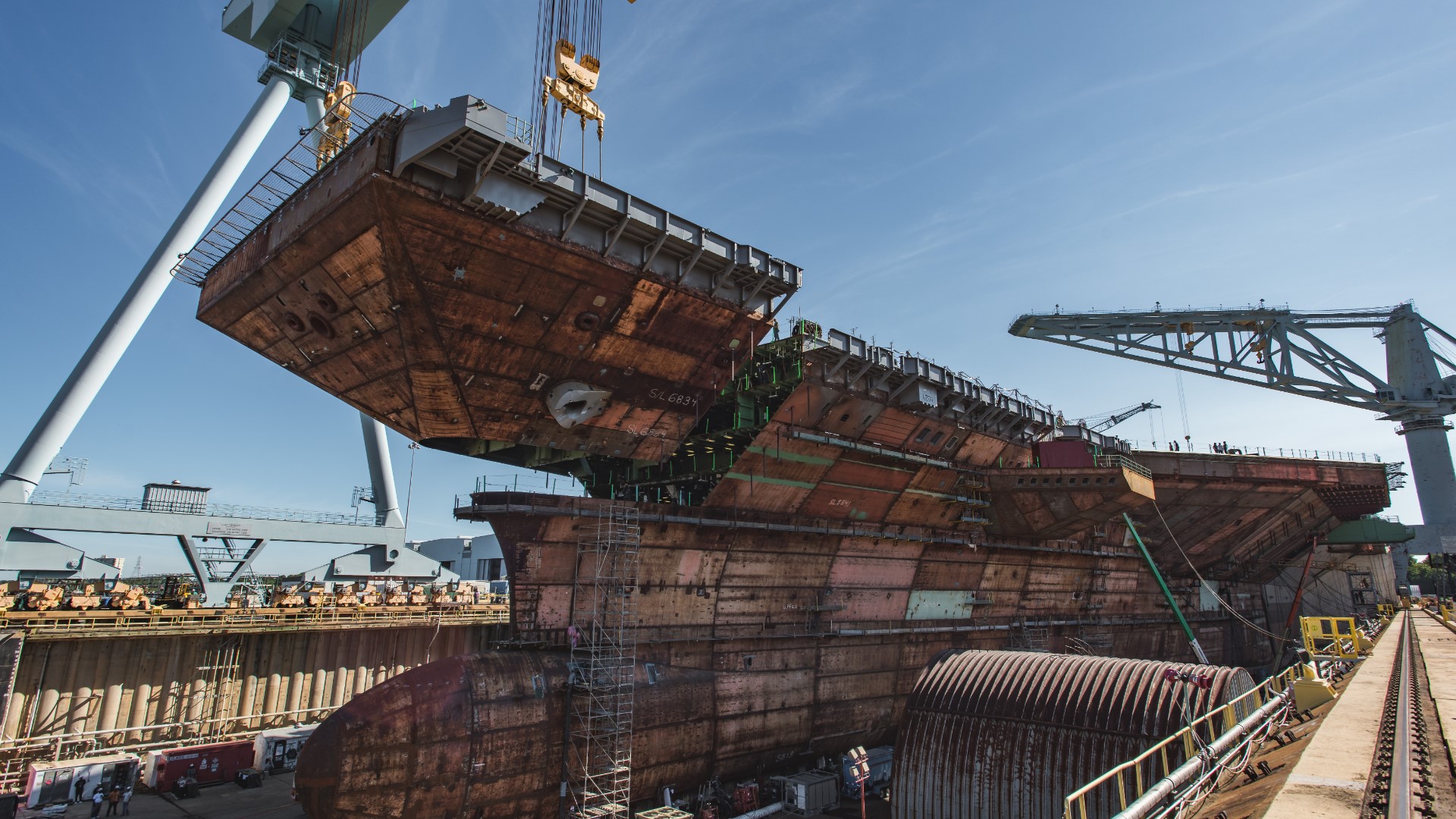The image depicts a massive, open-air shipyard on a clear, blue day. At the center lies an old, rusty ship, held upright by cranes and large cables. The ship's brown, deteriorated exterior suggests it has been weathered by time, and it seems to be either under construction or disassembly. Surrounding the ship are numerous industrial structures, including gray and light brown cranes, walkways, and scaffolding extending up the sides of the ship. In the lower-left corner, there appear to be train cars likely used for shipping purposes. The heavy-duty equipment and overall appearance of the yard support the conclusion that this is a photograph of a bustling, industrial port area.